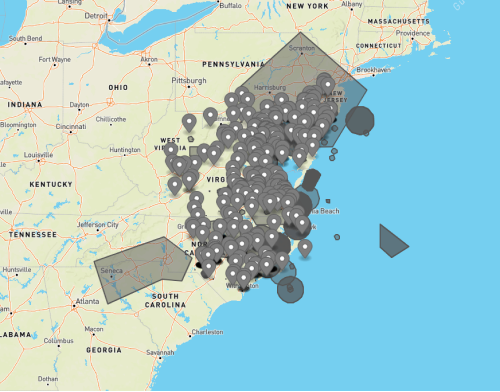This detailed map displays the northern part of the East Coast of the United States. The landmass is depicted in yellow, contrasting against the blue coloration of the water bodies. Prominent among the features are clusters of gray pointed circles that mark various significant locations on the map.

Starting from the northeast, the map includes the states of New York, Massachusetts, Providence, and Connecticut. To the west of Connecticut lies Pennsylvania, with Ohio positioned to its lower left. Additionally, south of the cluster of highlighted locations, South Carolina and Georgia are also mapped out.

The states and their relative positions are clearly delineated, with the clusters of gray and white pointed circles providing a focal point, indicating specific areas of interest within these regions.